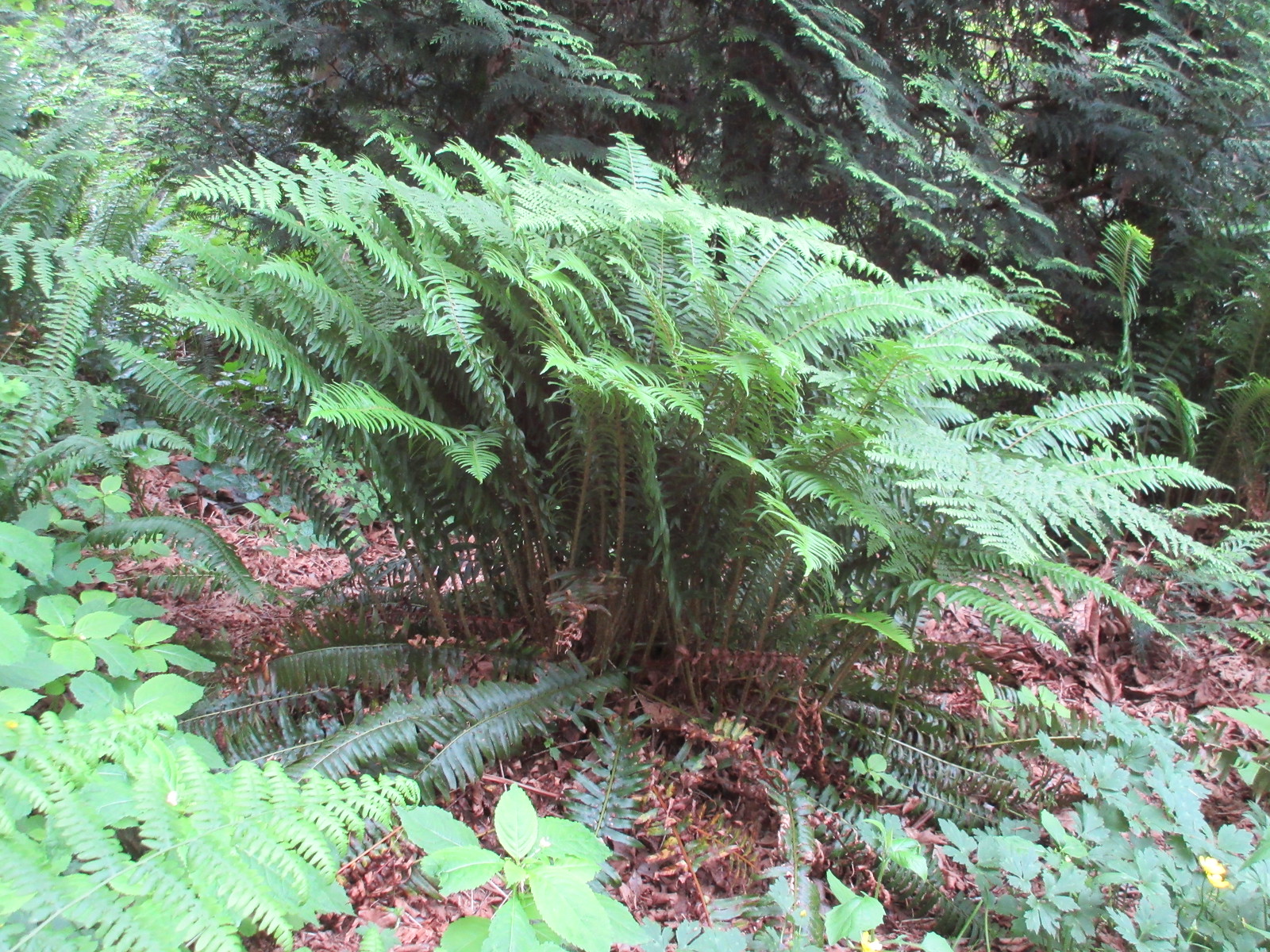This detailed photograph captures a lush outdoor scene, likely taken on a sunny summer day in a mildly wooded area. The focal point of the image is a verdant bush in the foreground, showcasing numerous thin, green leaves, suggesting a type of fern or a tropical plant native to forested environments. Surrounding the bush are various other green plants and foliage, with a hint of pink hues in some leaves, adding a splash of color to the predominantly green landscape. The ground beneath is scattered with dead or mulched leaves, lending a natural texture to the scene. The background features an array of trees, including pine and several other varieties, their presence casting sporadic shadows that confirm the bright daylight. A couple of vines can be seen climbing around the area, completing this vibrant, summery snapshot of nature in full bloom.